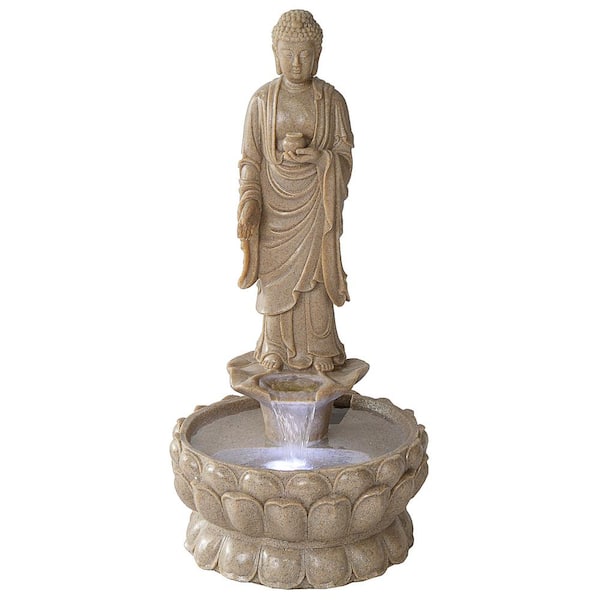The image depicts a detailed home decor item set against a white background. Central to the scene is a tan or brown statue of Gautam Buddha, characterized by a serene expression and dressed in a flowing robe with a headdress or cap. The Buddha statue stands on a rounded platform from which water cascades into a small, spherical fountain bowl. The bowl is adorned with decorative lotus or clamshell patterns that are evenly distributed around its exterior. There is an embedded light inside the bowl, illuminating the water as it pours. The Buddha statue is depicted in a barefoot stance, with one hand holding a cup, exuding a tranquil ambiance. The entire piece exudes an aura of tranquility, likely designed for home decor or as a gift item.